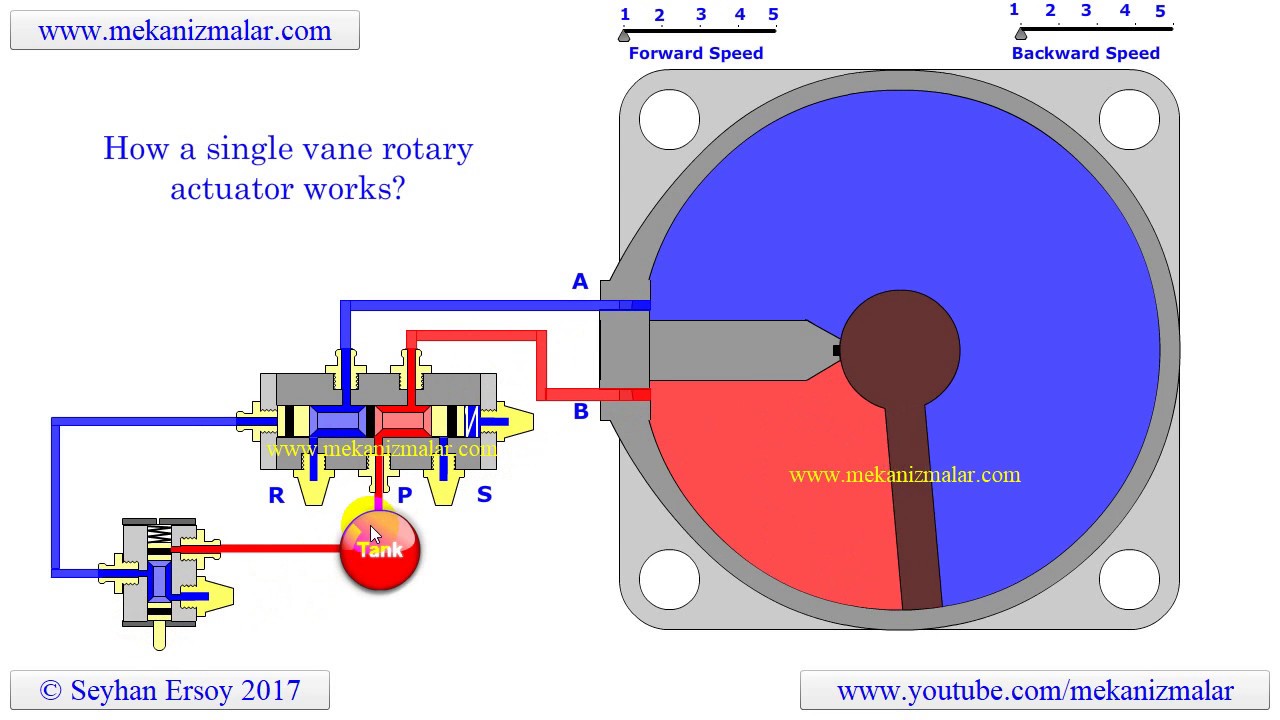The diagram in the image is set against a predominantly white background, which occupies most of the space. In the upper left-hand corner, there is a gray bar featuring blue text that reads "www.mechanizmalr.com." Below it, slightly to the right, a bold title poses the question, "How does a single-vane rotary actuator work?" 

To the right of this title, the diagram begins. Starting at the bottom left, a red circle labeled "Tank" is connected to a circuit featuring red and blue lines. The red line extends towards the left, while the blue line moves leftward, then upward, and finally to the right, leading to a gray rectangle. This rectangle contains colored components and diodes labeled "R," "P," and "S." A red line from the "P" diode heads towards the red circle labeled "Tank." Additionally, there are diodes on top of and to the right of the rectangle, each linked by lines: a blue line going up and right from the left top diode, and a red line going up, then right, then down from the right diode. 

These lines enter the next part of the diagram where the blue line is labeled "A" and the red line is labeled "B." They both converge into a circular section that is three-quarters blue and one-quarter red, with gray and white circular elements situated above, below, and on either side. In the center of this section, a dark brown circle with a protruding arm that extends downwards and to the right is visible. Below this circle, "www.mechanicular.com" is inscribed. 

Above the circular section, on both the right and left sides, there are meters labeled "Forward Speed" and "Backward Speed," each with indicators ranging from one to five. In the bottom right-hand corner of the image, there is a light gray bar displaying "www.youtube.com/M-E-K-A-N-I-Z-M-A-L-A-R" in blue text. Additionally, "Copyright Sehan Ersoy 2017" is noted in blue text, adding a final touch to this detailed and intricate diagram.